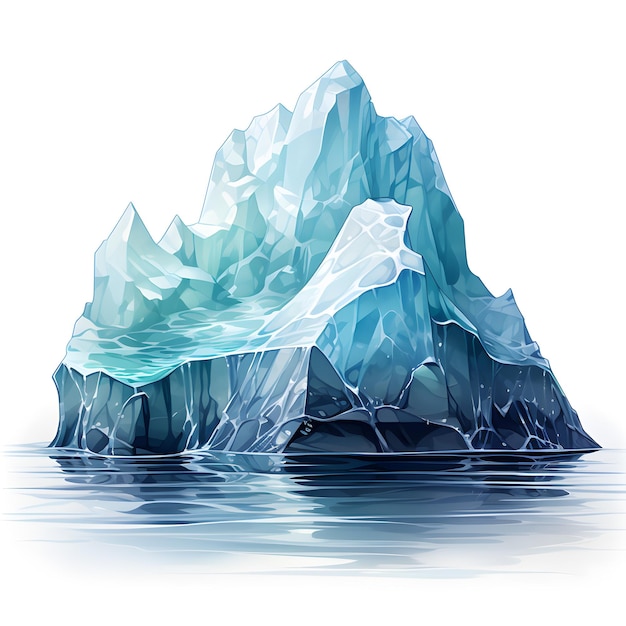This image, rendered in a graphic, cartoonish style, depicts a striking illustration of a triangular-shaped glacier floating in the ocean, set against a completely white background, devoid of text. The glacier's base is a deep, dark blue, transitioning to a lighter blue as it rises, culminating in a jagged, white-tipped peak. The glacier features multiple pointed peaks, adding to its dramatic appearance. Below the glacier is a calm body of water, displaying a mix of white and light blue hues, with reflections of the dark blue base enhancing the depth and serenity of the scene. The ocean surface is mostly still, with no white caps, creating a tranquil yet stark contrast with the rugged, icy formation above.